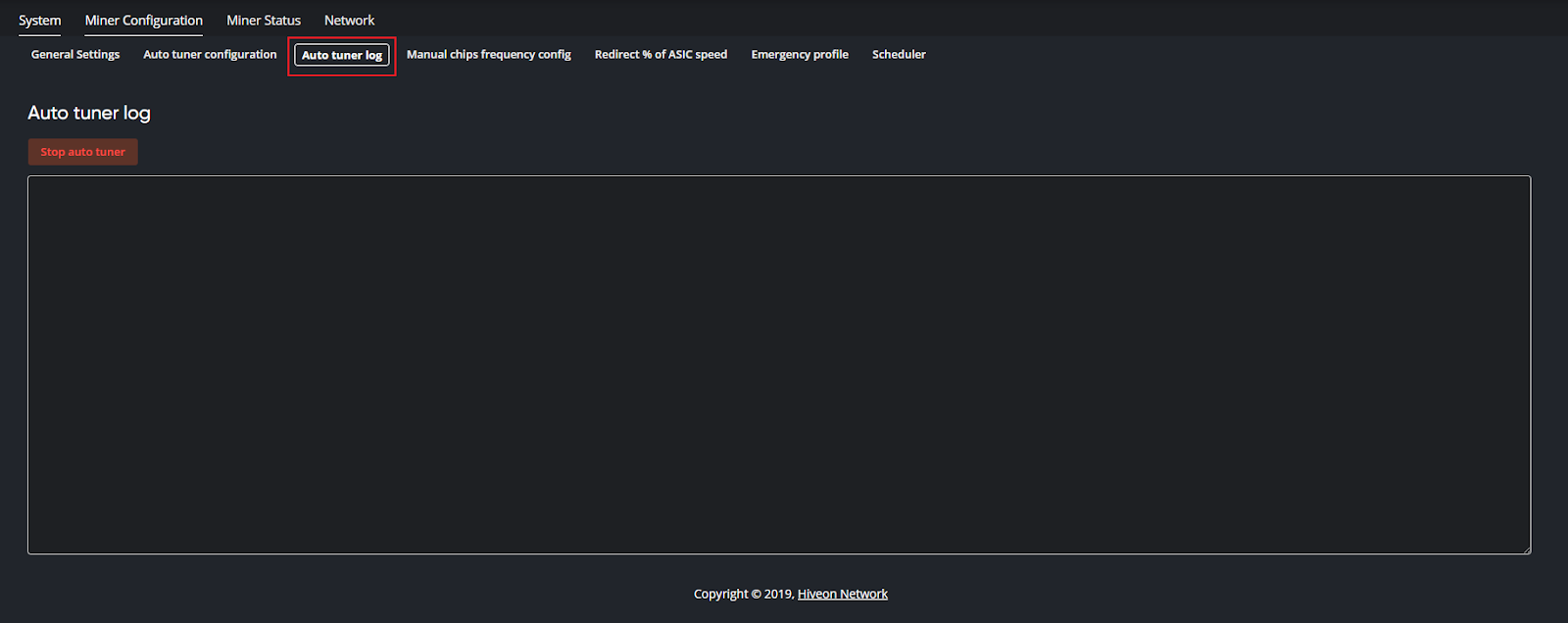The image depicts a website designed with a dark black background. At the top, prominent white text reads "System" with an initial capital 'S,' and it's underlined by a white line. Adjacent to it is the section titled "Miner Configuration," where both words are capitalized and underlined in white as well. Following this, there are labels for "Miner Status" and "Network."

Further down, the website displays several navigation options in white text, including:
- General Settings
- Auto-Tuner Configuration
- Auto-Tuner Log
- Manual
- Chips Frequency
- Coding
- Configuring
- Redirect
- Percentage of a CIC
- Speed
- Emergency Profile
- Scheduler

Proceeding lower on the page, there’s a label "Auto-Tuner Log" alongside a red banner that reads "Shop Auto-Trader" in bright red text.

Towards the bottom of the image, a rectangle with a black border encloses more white text, and at the very bottom, the footer text states, "© 2019 Hivion Network," where 'Hivion Network' is capitalized, with 'H' and 'N' distinctly highlighted.

Overall, the design of the page is sleek with a high-contrast color scheme primarily using black and white, accentuated by occasional red elements for emphasis.